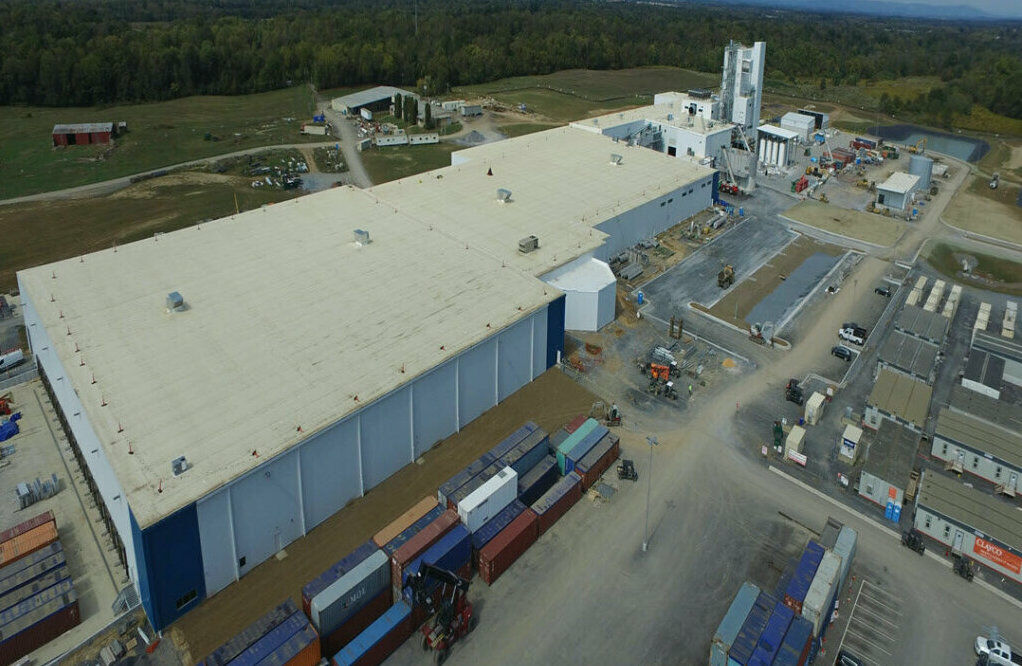This is an aerial photograph of a large industrial warehouse with a light-colored, flat roof featuring five silver fans. The warehouse, characterized by its modular, rectangular, and flat-walled design with gray and blue corners, extends across the image from the left side to the upper right part. Surrounding the warehouse are approximately 25 multicolored shipping containers, including shades of blue, maroon, orange, and light blue. Adjacent to the warehouse is an industrial plant and a massive parking lot with a few trucks. Bordering the scene are green trees and wooded areas, while the sky appears dark and overcast, suggesting imminent rain. In the upper left corner, a barn-like structure is visible, adding to the diverse industrial landscape depicted.